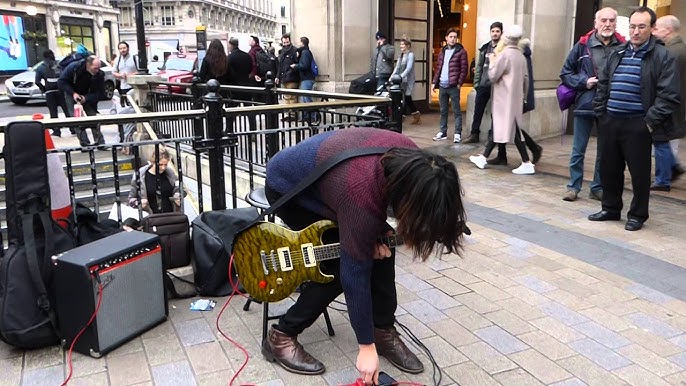In this detailed image set in an old downtown area, a long-haired guitar artist wearing a colorful purple and blue sweater is the focal point. He holds a dark gold electric guitar connected to a grey amp on his left, appearing to adjust his musical gear. The scene is bustling with people gathered and chatting, some of them watching him intently. The stone-paved area, flanked by stone brick streets and a walkway, hints at a European setting. In the background, stairs suggest access to a subway, while a few cars drive along the distant road. Despite the busy surroundings, the artist captures the moment with his imminent musical performance.